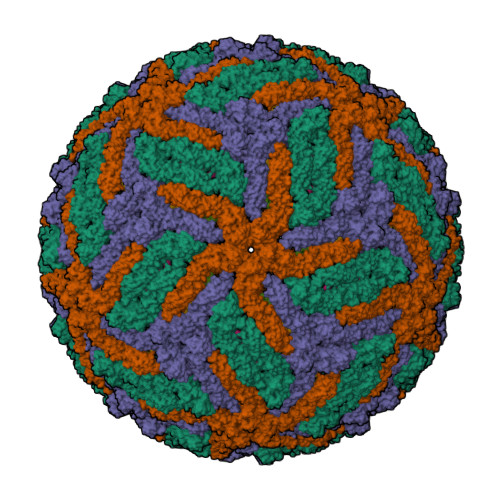In this detailed image, the focal point is a large, textured spherical object predominantly crafted from what appears to be clay. The ball features an intricate blend of colors, including shades of orange, turquoise, purple, and deep red. At the very center, there is a tiny white dot from which an orange spiral pattern emanates, giving the impression of elongated star-like arms stretching outward. This spiral design is interspersed across the sphere, creating a striking visual effect. Complementing the spiral patterns are rectangular aqua blue patches and three-pointed purple shapes that fill in the remaining spaces. The surface of the ball is notably textured, resembling coral with its rough, clumpy, and jagged appearance. Set against a simple white background, the ball's vibrant and complex design stands out distinctly, making it the unquestionable centerpiece of the photo.